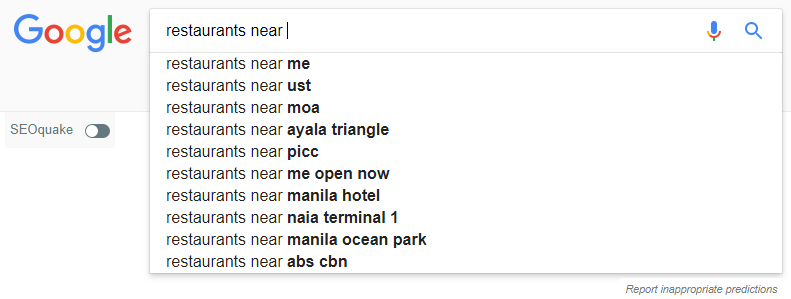The image is a screenshot of the Google search engine homepage. Prominently displayed on the left side is the iconic Google logo, composed of a sequence of colorful letters: a blue "G," followed by a red "O," a yellow "O," a blue "G," a green "L," and a red "E." Directly beneath the logo, in a small gray font, is the text "SEOquake," accompanied by a small line with a circle and half-circle icon. SEOquake is identified as a browser add-on tool useful for keyword research.

Centered on the page is the search box, which contains the partially typed query "restaurants near." Displayed below the search input field is a dropdown list featuring related search suggestions:

1. Restaurants near me
2. Restaurants near USTMOA
3. Restaurants near Ayala Triangle
4. Restaurants near PICC
5. Restaurants near MeOpenNow
6. Restaurants near Manila Hotel
7. Restaurants near NAIA Terminal 1
8. Restaurants near Manila Ocean Park
9. Restaurants near ABS-CBN

The dropdown provides various localized search options to assist users in finding nearby restaurant locations based on specific landmarks and areas in Manila.